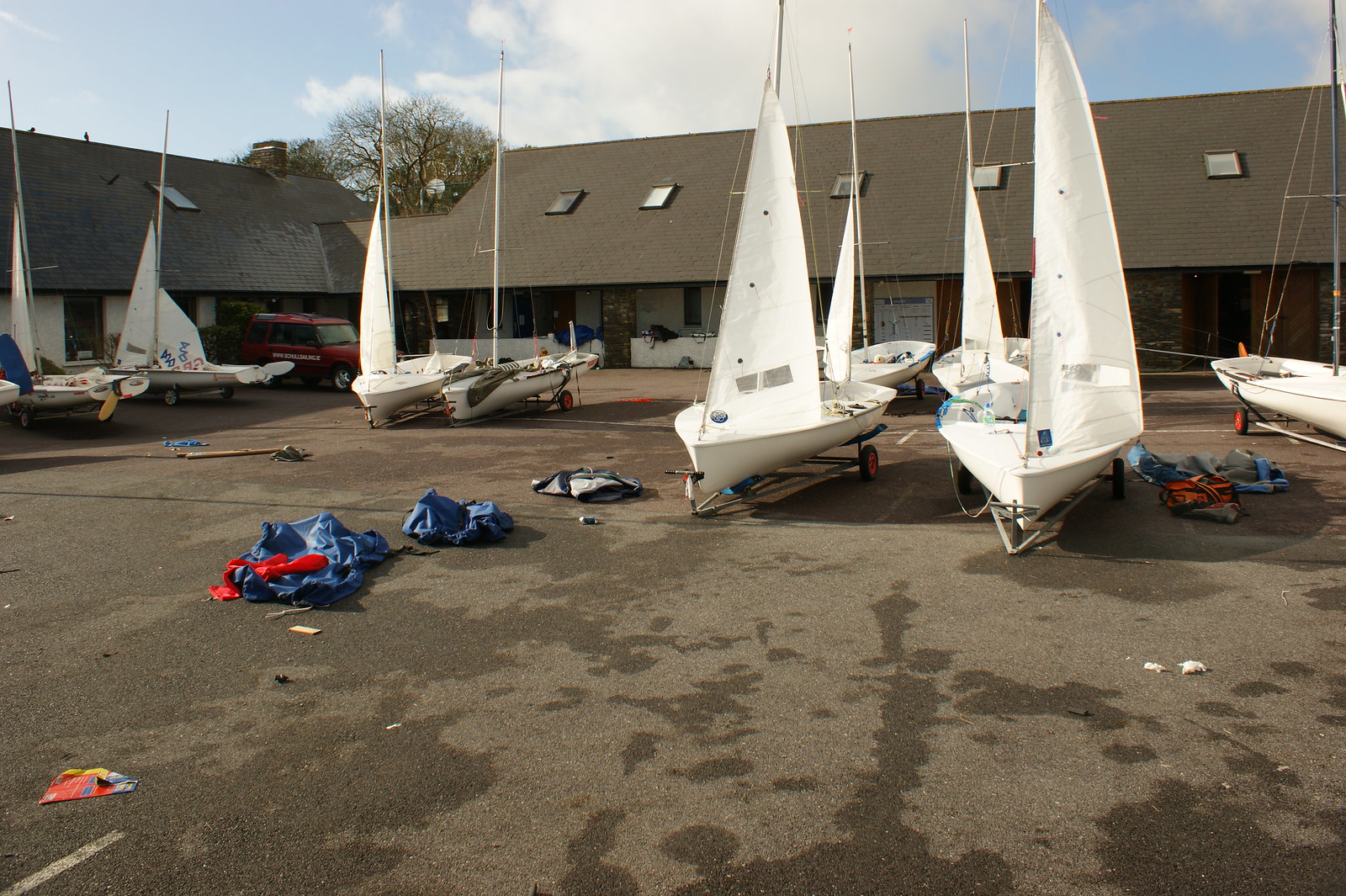This photograph captures a lively scene in the parking lot of an office building complex with a high gable roof, likely a motel or a beach town facility. The buildings feature external doors and numerous skylights. Instead of cars, the lot is filled with at least nine sailboats, each white with matching white sails, all perched on trailers with wheels. The ground around these boats is dotted with neon bright orange life jackets and blue boat covers, suggesting recent or ongoing activity. A solitary red jeep, bearing an unreadable logo, is parked in the background. The scene is bathed in natural light, with a clear blue sky, a single white cloud, and a green tree visible between the structures. The damp, mottled appearance of the ground hints at recent rainfall, adding to the vibrant and dynamic atmosphere of the image.